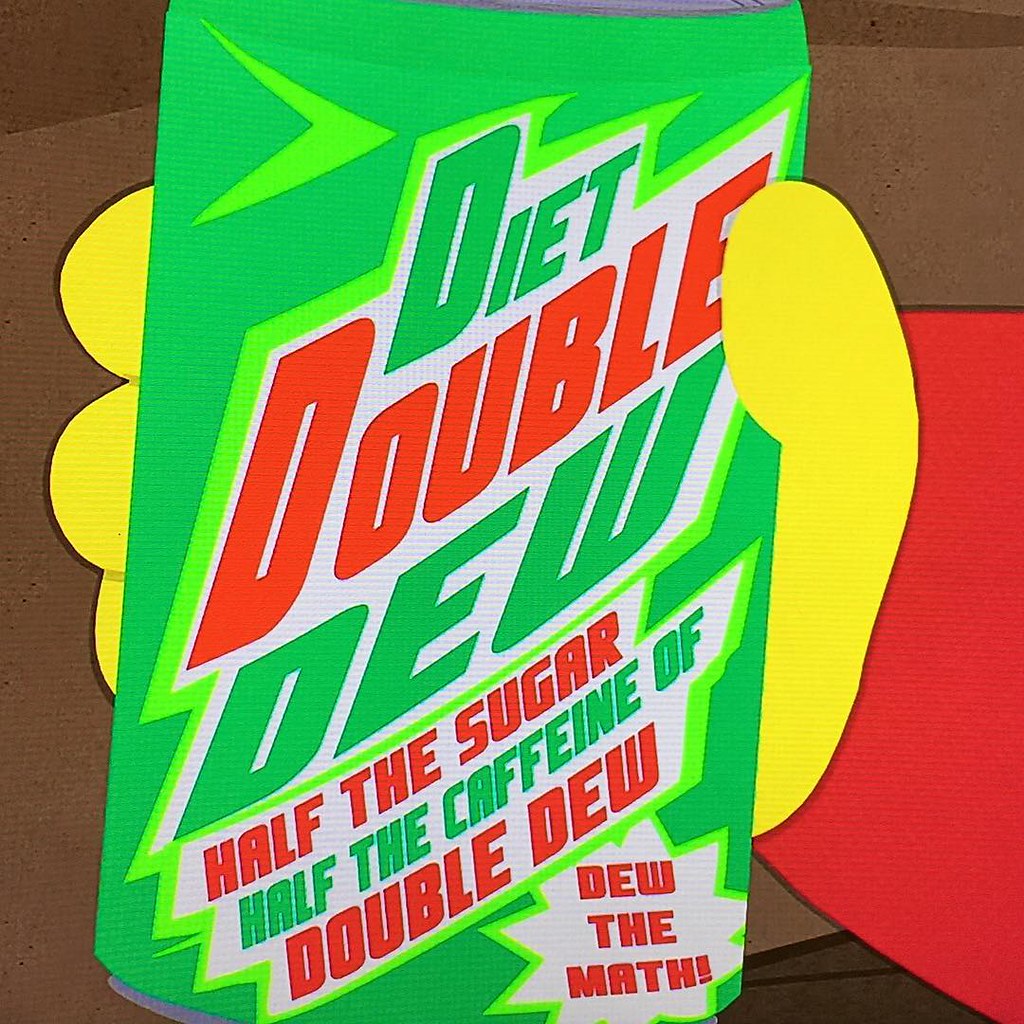The image is a square, digital cartoon illustration featuring a stylized yellow hand with four fingers (including the thumb) gripping a green soda can, partially obscured at the top and bottom. The hand, emerging from a bright red sleeve, prominently displays three fingers wrapping around the left side of the can, with the thumb visible in the foreground on the right. The can, mimicking the branding of Mountain Dew with a similar color palette of silver, dark green, light green, and red, is labeled "Diet Double Dew." The text layout presents "Diet" in green, "Double" in red, "Dew" in green, and a silver-grey background for the text. Additional text on the can reads "half the sugar, half the caffeine of Double Dew" and "Dew the Math!" in red font. The image is set against a brown background, highlighting the vivid colors and playful design of the hand and can.